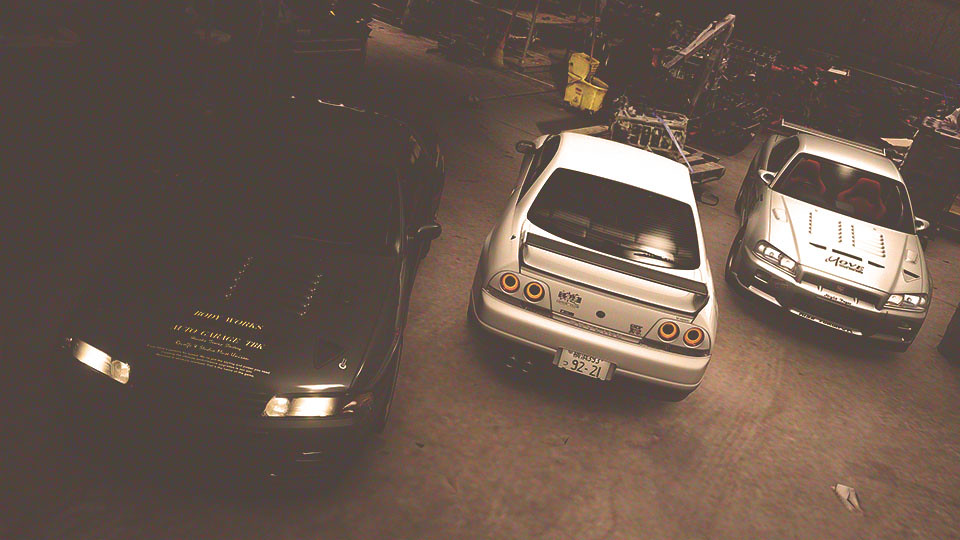The photograph, taken at night or in a dimly lit environment, depicts three vehicles parked in what appears to be a large mechanic's garage, illuminated by artificial lighting. To the left, there is a black Nissan Skyline with its headlights on and gold writing on the hood; it seems to be a two-door model. In the middle, a silver two-door Nissan Skyline GT-R is positioned with its rear end facing the camera, featuring a large wing and Japanese license plate writing. The right-most vehicle is another silver Nissan Skyline, heavily customized with hood vents, red seats, aftermarket mirrors, and a large wing, facing the camera. The garage is well-equipped with an engine hoist, toolboxes, workbenches, and various machinery in the background. Notably, a big yellow mopping bucket and a wooden crate with an engine block on top are located near the middle car.